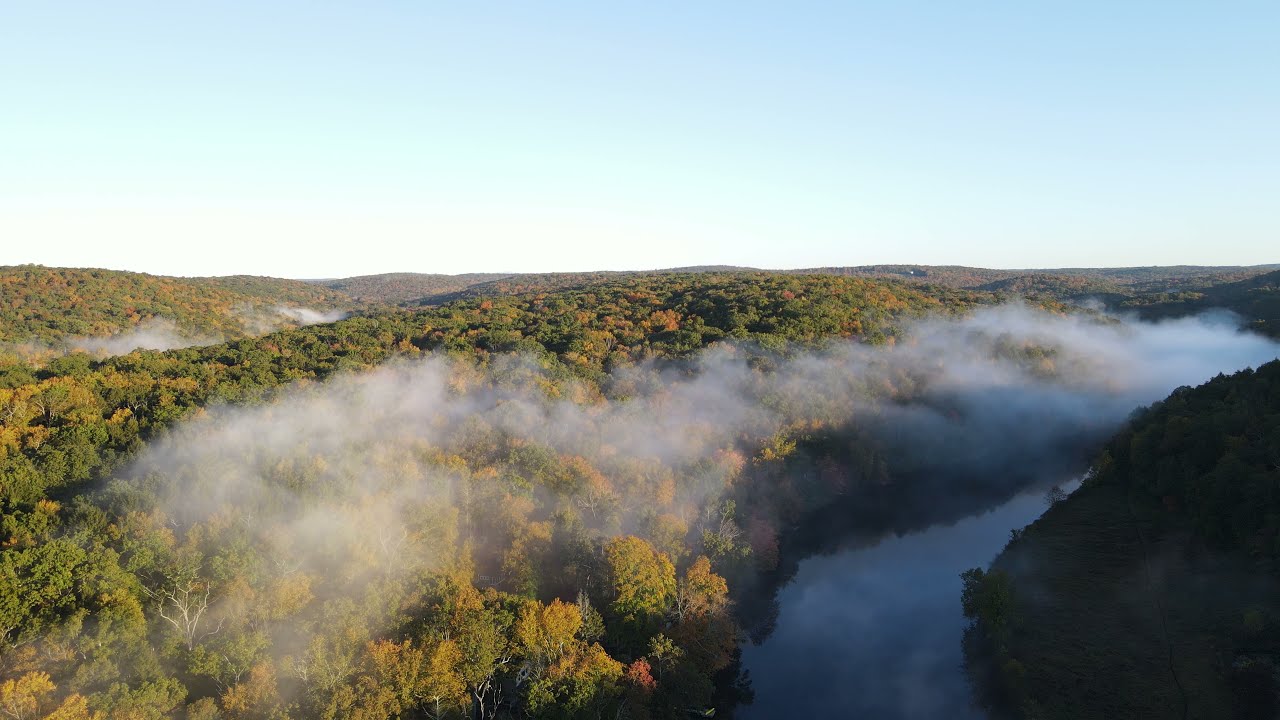The full-color outdoor photograph, likely taken in early fall, captures a serene, high-altitude view from possibly a tower, drone, or helicopter during the daytime. Dominating the upper third of the image is a bright blue sky with a few wispy clouds scattered near the horizon. Below, the majority of the scene showcases lush, rolling hills or mountains densely covered with green trees beginning their transition into the yellow hues of fall. Between these hills, pockets of thick white fog, perhaps from a nearby river seen on the lower right in shadow, rise and wisp through the landscape. This early morning scene, steeped in mist and shadow, paints a tranquil picture of the changing season in a forested area, hinting at the river's contribution to the misty ambiance.